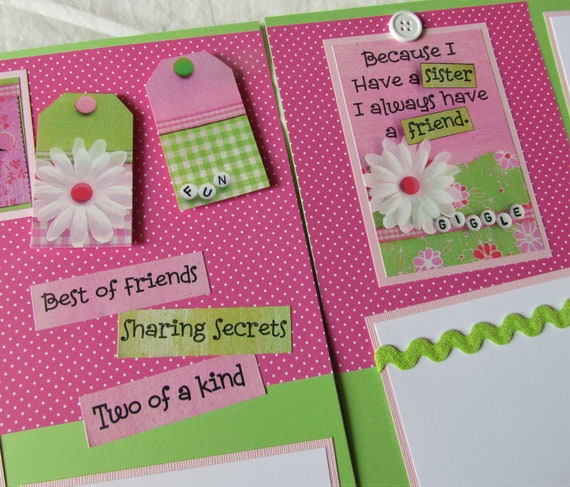This image portrays a pair of vibrant, cheerful scrapbook pages. The background features a playful contrast of lime green and pink-with-white-polka-dots. A multitude of whimsical elements like flowers, buttons, and ribbons adorn the pages. The texts "Best of Friends," "Sharing Secrets," "Two of a Kind," and "Because I have a sister, I always have a friend" are prominently displayed on colorful slips, adding to the sentimental value of the scrapbook. Dainty white buttons spell out "FUN" and "GIGGLE," enhancing the playful and upbeat mood. The zigzagging green ribbon and daisies with red centers further accentuate the scrapbook's lively and friendly aesthetic.